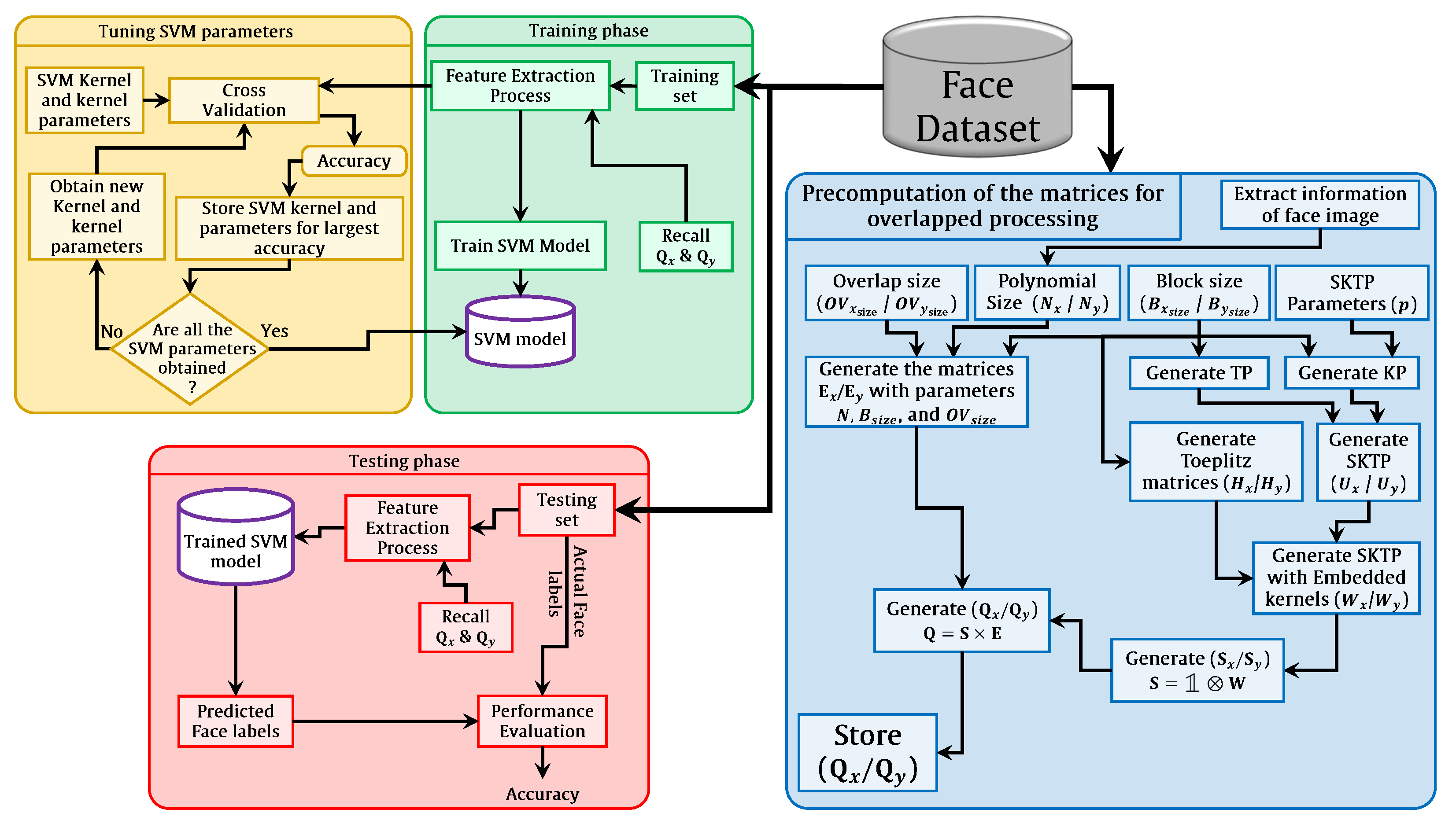This image is a detailed flow diagram related to facial data processing and recognition, divided into color-coded sections that represent various phases and tasks. At the center, a silver cylinder labeled "Face Dataset" acts as the primary data source. The process begins with a yellow box titled "Tuning SVM Parameters" which delves into setting up the support vector machine (SVM) for facial recognition. Following this, a green box labeled "Training Phase" involves extracting and processing face images to train the SVM model, incorporating scientific terms such as kernel parameters, cross-validation, and accuracy metrics. The diagram continues to a large blue box named "Precomputation of the Matrices for Overlap Processing," which deals with the computational setup required for analyzing the data. Finally, a red box at the bottom left titled "Testing Phase" outlines the steps for validating the trained model, including decision-making processes represented by yes/no paths and algebraic expressions. Arrows connect these stages, forming a coherent and interconnected grid that systematically outlines the entire facial recognition workflow.